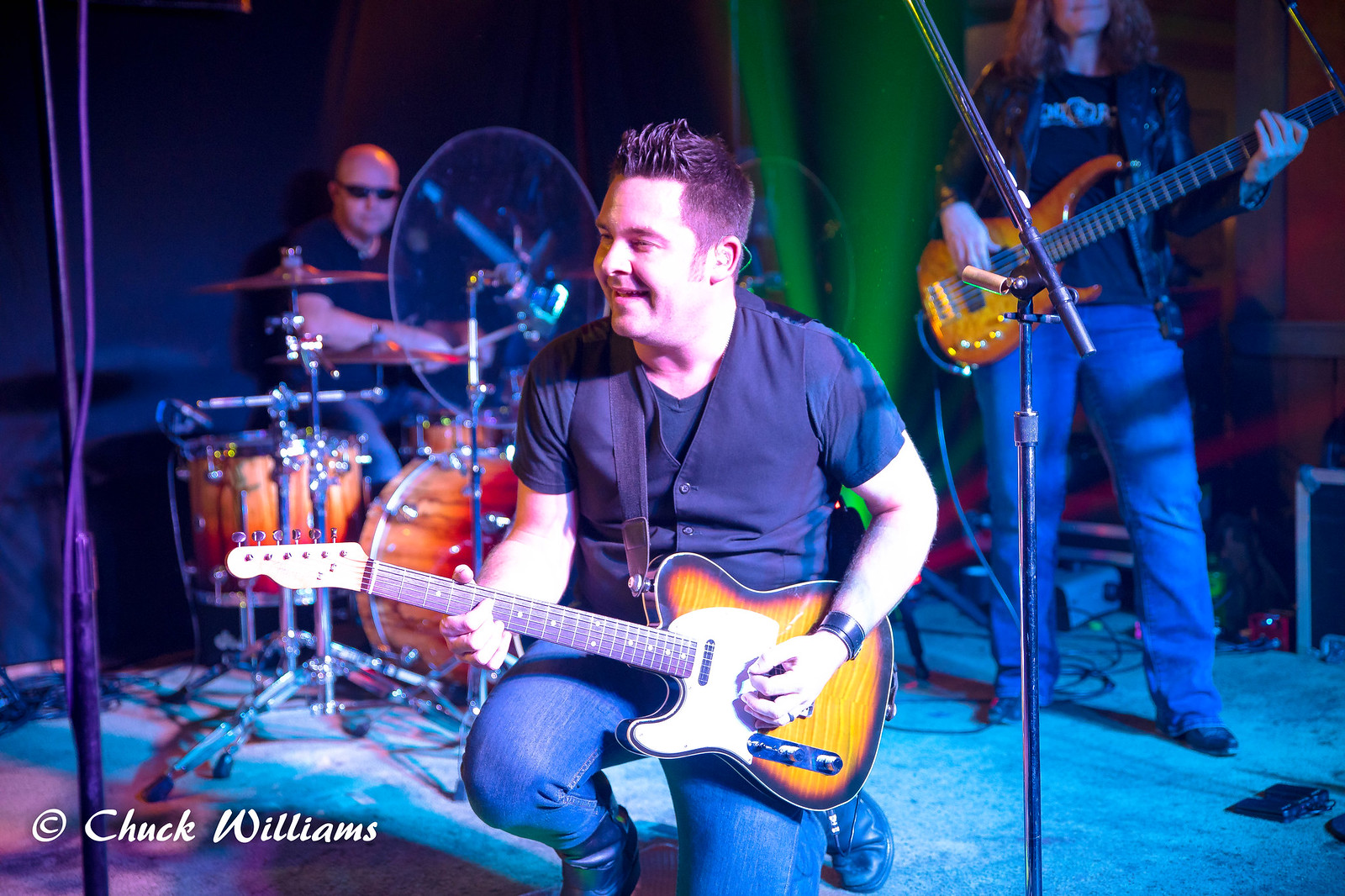In this wide rectangular image, a band is performing on a carpeted stage with a blue tint on the floor. The focal point is a man kneeling in the center, facing slightly to the left. He is a white male with spiky brown hair, wearing a dark blue t-shirt and a buttoned dark blue vest, along with blue jeans and dark shoes. He is playing an electric guitar, smiling as he looks slightly diagonally. To his right and slightly behind him stands another band member in blue jeans and a black leather jacket, playing a similar electric guitar or bass. This individual wears a black t-shirt with white lettering and black shoes. To the left and behind the central figure is a bald, white man wearing sunglasses and a black t-shirt, seated at a drum set. The stage is illuminated with blue, green, and red spotlights creating strobe light effects, and a green curtain along with a black backdrop can be seen behind the performers. Text at the bottom of the image reads, "Copyright Chuck Williams" in white.